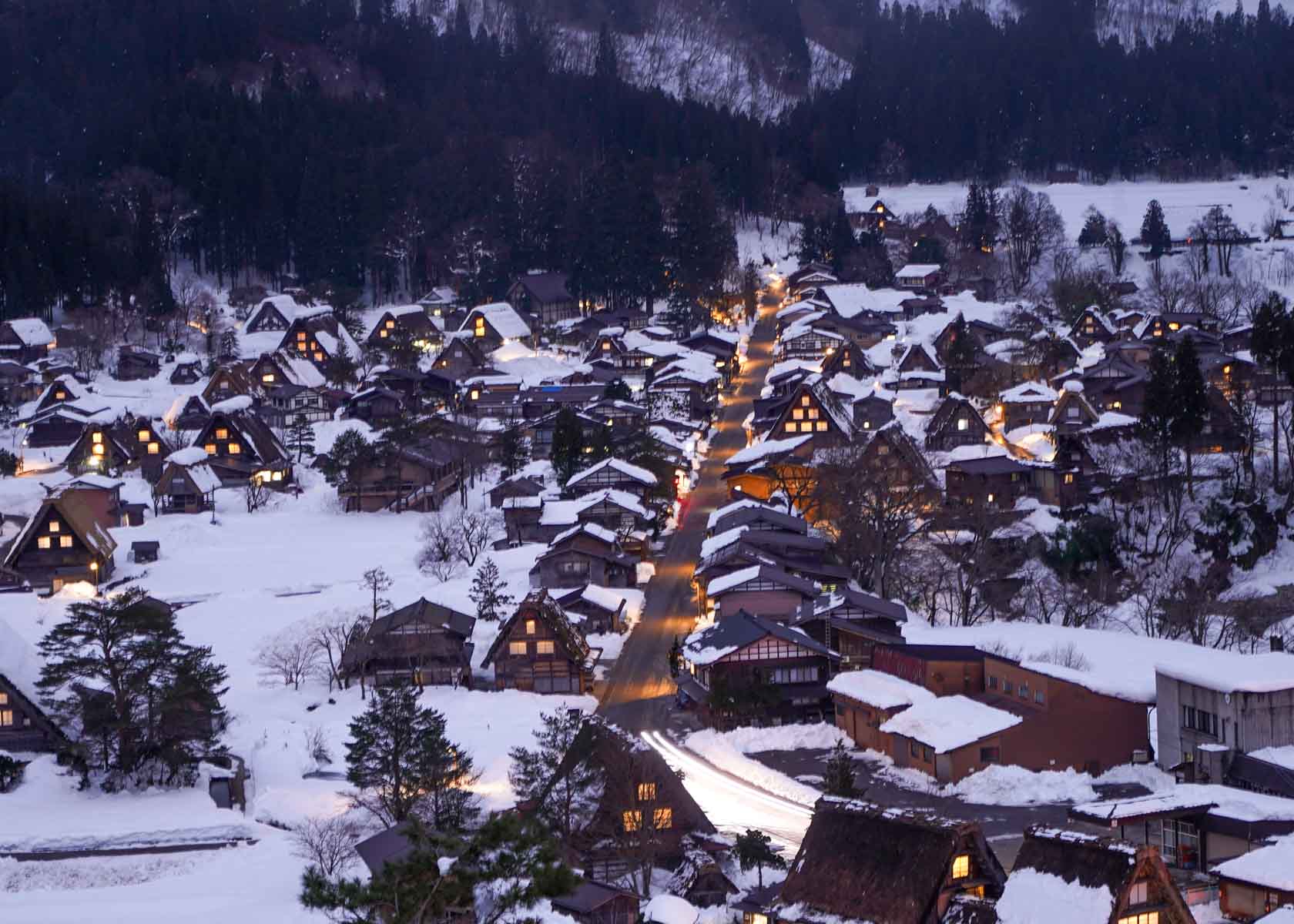This image captures a picturesque, almost square, outdoor landscape scene. The top portion features a range of hilly mountains adorned with dark pine trees and lighter green trees, interspersed with patches of snow visible through the bare branches. Below the mountainous terrain stretches a charming mountain village occupying approximately three-fourths of the photo. The village is crisscrossed by a road that winds down from the center to the bottom and then veers to the right. The road has pockets of blown snow, though most areas remain clear. The town consists of numerous brown houses, many with V-shaped, pointed roofs, casting a cozy, rustic charm. Warm yellow lights emanate from the windows and street lamps, suggesting it is either early morning or late evening. On the right side of the village, there appears to be a body of water surrounded by trees, which might be frozen. Additionally, there are a few storefronts constructed from brown wood, seamlessly blending into the natural surroundings. The overall scene conveys a tranquil, wintery mountain atmosphere, peppered with signs of life and activity.